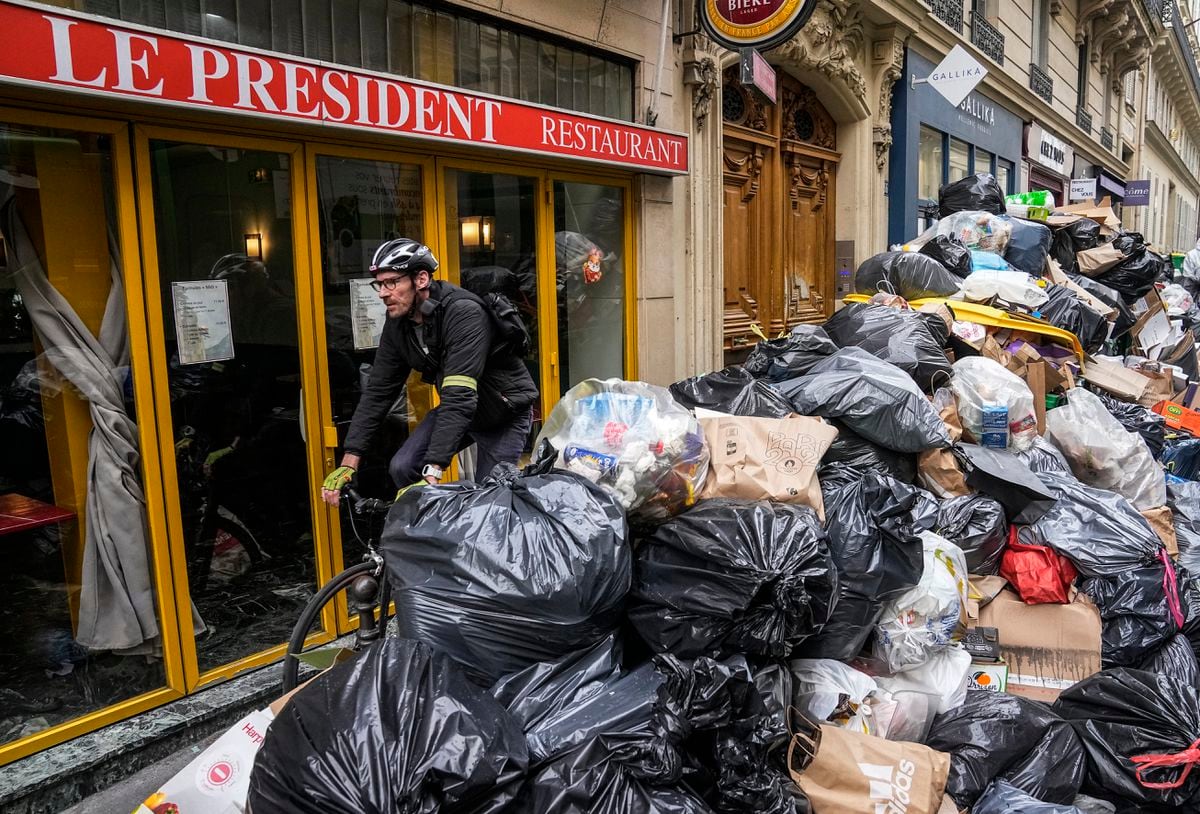In this striking photograph of a bustling city street, we are presented with a dramatic scene featuring "La Presidente" restaurant, distinguishable by its red background and white text signage. The street appears to be in the midst of a severe garbage strike, as an immense mountain of trash bags stretches as far as the eye can see down the sidewalk. The heap of refuse reaches an impressive height of six to seven feet, towering over a cyclist who navigates the narrow, congested path. Dressed in black biker gear with a black and white striped helmet and glasses, the cyclist maneuvers his black bicycle with great difficulty past the obstructing trash. The overwhelming pile of garbage, primarily in black hefty bags with some red and clear ones interspersed, spreads across an estimated 10 to 15 yards. Brick buildings and various storefronts loom in the background, offering a stark contrast to the chaotic accumulation of waste in the foreground.